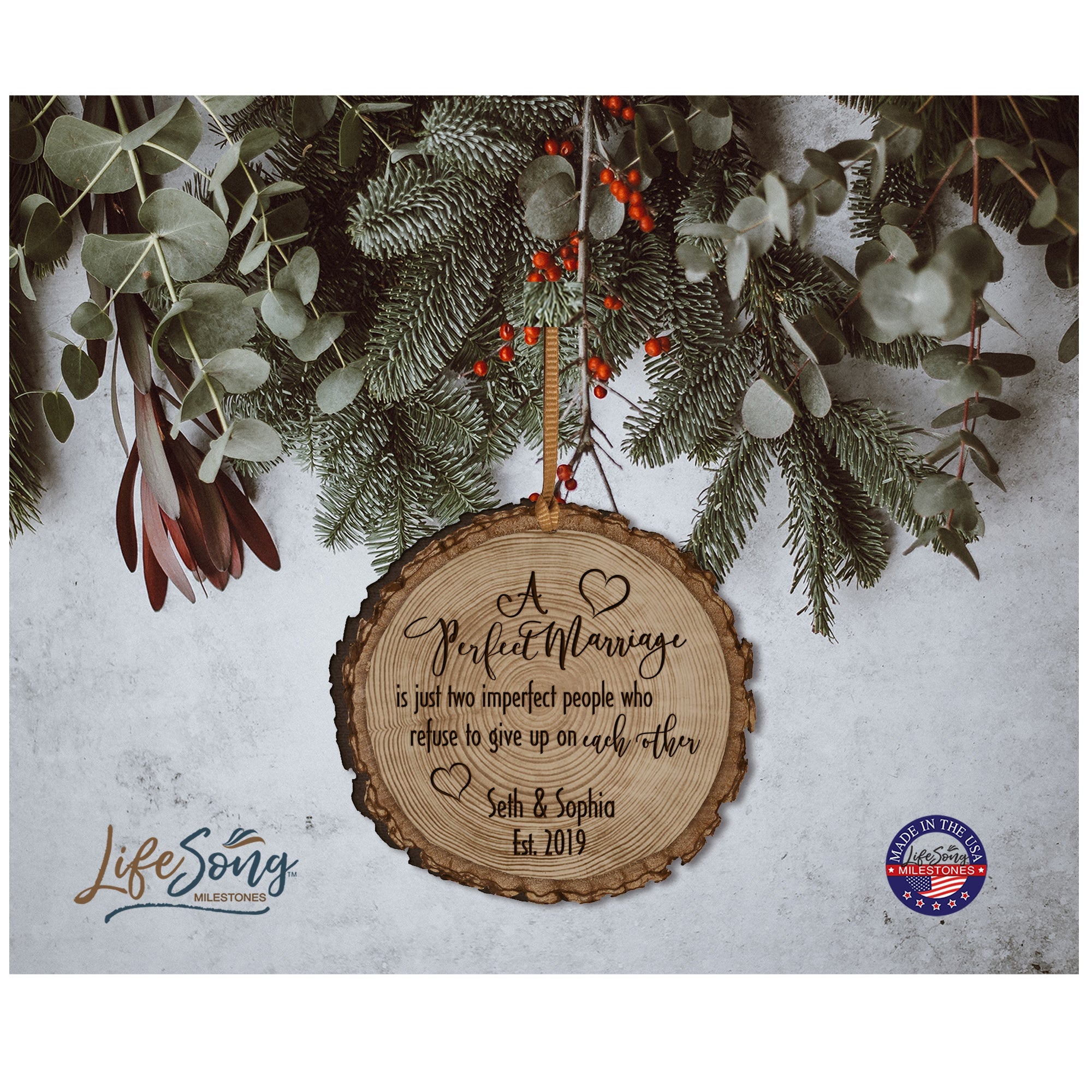The photograph depicts a rustic Christmas ornament made from a circular slice of wood, designed to look like a tree ring. The ornament is inscribed with the phrase "A perfect marriage is just two imperfect people who refuse to give up on each other," written in cursive. Above the word "marriage," there is a small heart. Below the quote are the names "Seth and Sophia" and "EST 2019." The ornament hangs from a piece of brown ribbon, amidst festive holiday greenery that includes spruce or pine branches, mistletoe, red berries, and leaves with whitish-green highlights. The background appears white, adding a wintry feel. In the lower left corner of the image, there is a logo that reads "Lifesong Milestones," while the lower right corner contains a "Made in the USA" emblem within a circle that features an American flag on the bottom half.